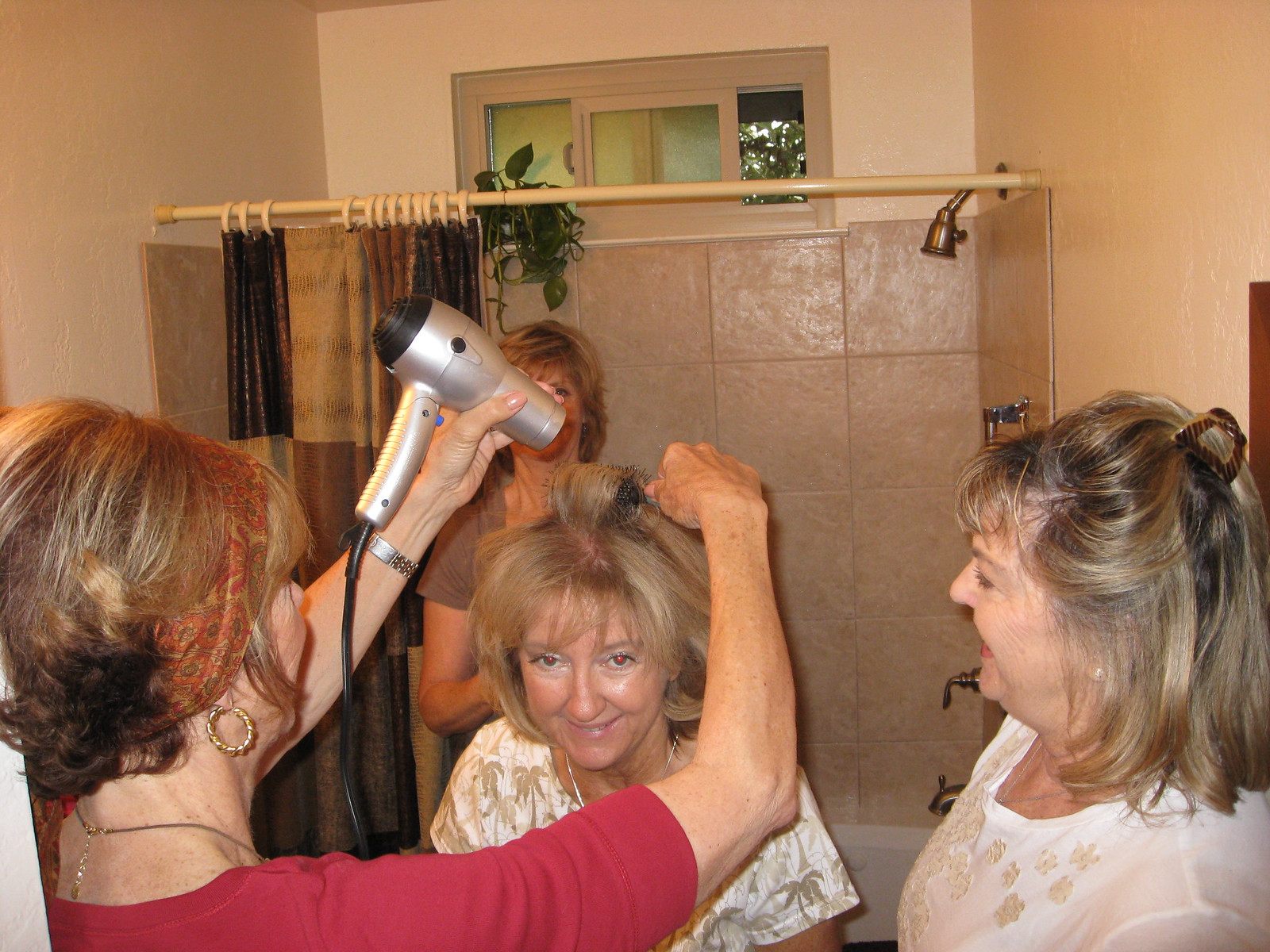In this detailed photograph, four women are gathered in a small bathroom with a beige and tan color scheme. An elderly woman, sitting in front of a white bathtub and partially obscured shower curtain with light-colored browns and blacks in a checkered pattern, is having her hair styled. She has light brown hair that cascades to her shoulders, deep blue eyes, and a warm smile. She wears a white blouse adorned with faint gold palm tree patterns, a delicate necklace, and a touch of pink lipstick.

Positioned to the bottom left, another woman with short, light brown hair styled in a floral-themed headband is focused on blow-drying a curled section of the seated woman's hair. She is dressed in a reddish-pink top that reaches her elbows. She sports small gold hoop earrings, a gold necklace, and a metallic watch on her left wrist while handling a silver hair dryer and round black brush.

Behind the woman doing the blow-drying, partially blocked by the hair dryer, is a third woman with shoulder-length blondish-brown hair, clad in a brown top. Her face is not visible due to her position. To the right side of the image, a fourth woman with short blondish-brown hair pulled up with a barrette is watching the hair styling. She’s wearing a white dress with small appliques.

The bathroom's decor includes a shower curtain rod with matching beige rings and a green plant visible through a small, three-paned window above the bathtub. The walls and large tiles in the shower area are all shades of beige, complementing the serene and warm atmosphere where this intimate moment of care and companionship unfolds.